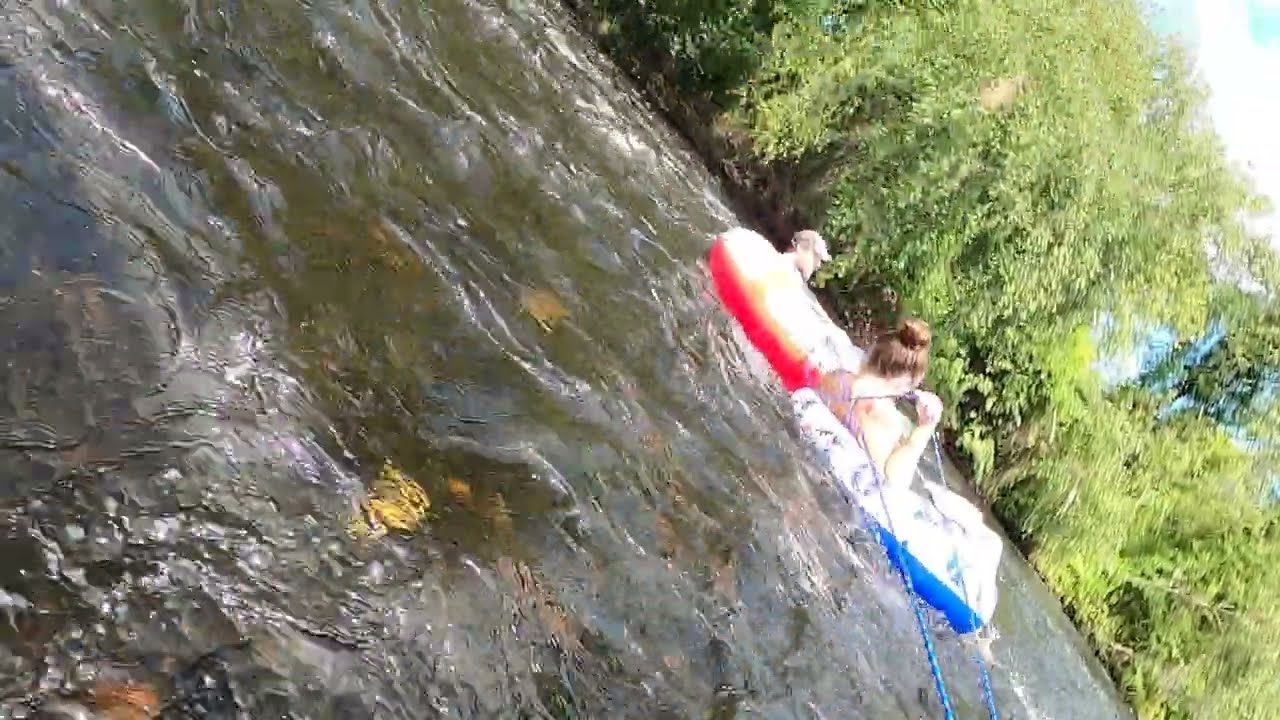This photorealistic but low-resolution image depicts an outdoor scene of a river with two people floating on it, using flotation devices. The photograph appears to be taken at a diagonal angle, with the river's surface extending from the center of the top part of the image down to near the bottom right corner. The water has a greenish-brown hue, appearing more transparent close up, and contains floating yellow and brown debris. Surrounding the waterline is abundant foliage including tall trees and various plants in bright and dark greens.

Just to the right of the image's center, we can see a woman and a man floating leisurely. The woman, who is positioned more towards the right, has brown hair pulled up in a bun and is lying on a white and blue flotation device. She is holding a blue rope that stretches off the screen towards the bottom of the image. Adjacent to her and slightly behind, the man is wearing a hat and sitting on a white and red flotation device. The serene scene suggests they are enjoying a lazy, sunny day on the river, with calm, slowly flowing waters and no signs of rapids. The photographer seems to be in the river with them, capturing this tranquil moment.